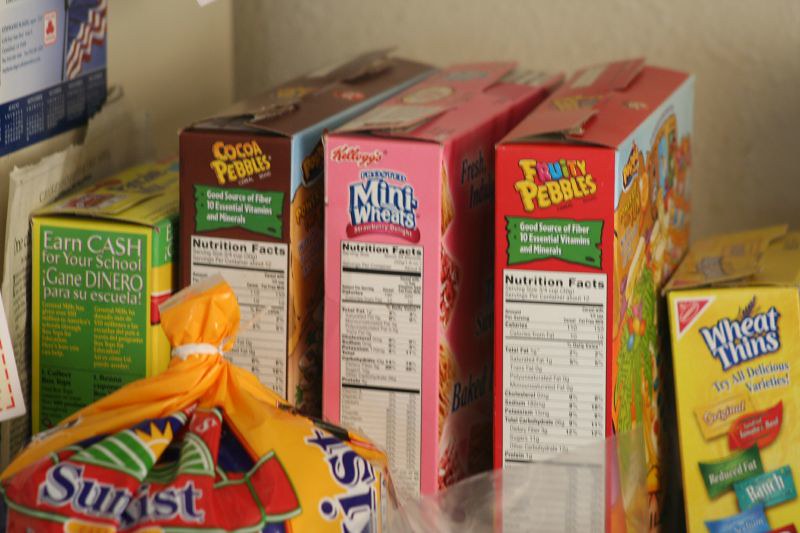The image depicts a collection of food items arranged against a wall. Prominently featured in the center are three cardboard boxes of cereal, each positioned with their nutrition labels facing forward. To the left of these cereal boxes sits a shorter, non-cereal cardboard box, while on the right, a box of Wheat Thins is clearly visible. In the forefront of the arrangement is a sealed bag of Sunkist snacks, identifiable by a distinctive white band securing its top. The items are neatly leaned against the wall, which itself has various objects attached to it, providing context and a sense of the environment in which these food products are placed.